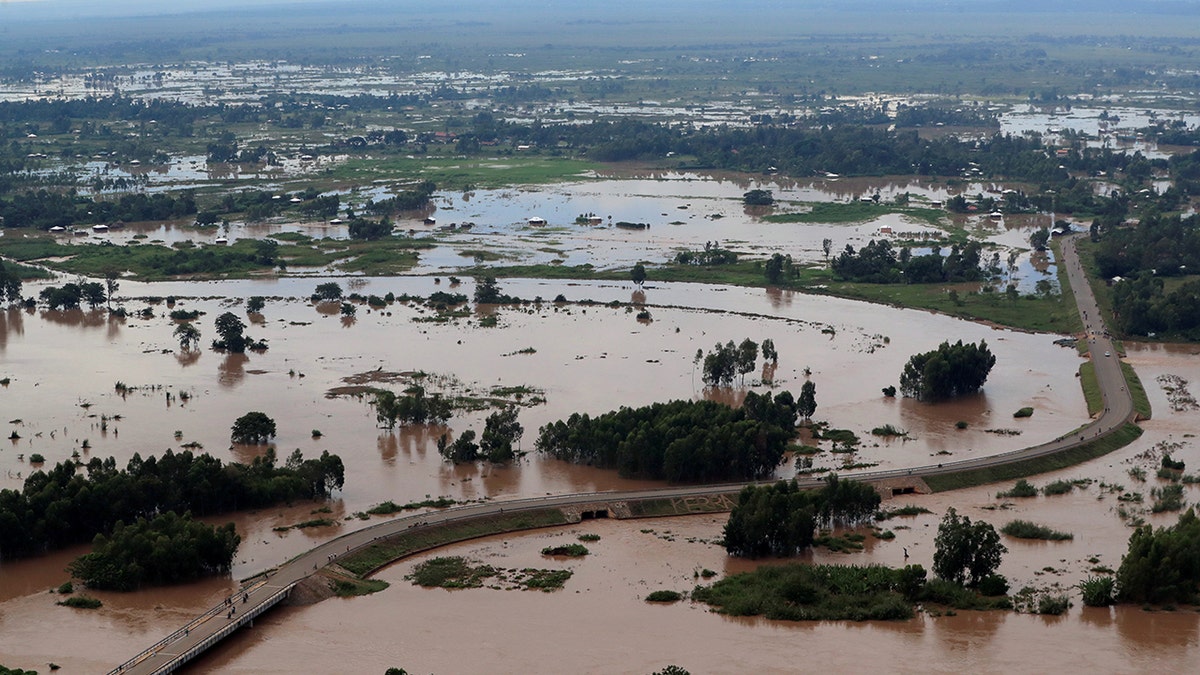The image reveals an aerial view of a sparsely populated, flood-affected landscape taken from an elevated angle. Predominantly featuring natural scenery with scattered trees and patches of greenery, the scene extends into the far horizon. In the foreground, brown floodwaters inundate vast areas of land, partially submerging trees and houses, with some structures appearing halfway underwater. A prominent winding road, which seems to be a highway, cuts through the scene, elevated above the floodwaters. There is a bridge starting from the lower left corner, curving to the right and then stretching straight upwards, teeming with people walking across it, but no visible cars. In the distance, more flood-stricken land and scattered homes and trees can be seen, underscoring the extensive impact of the flooding.